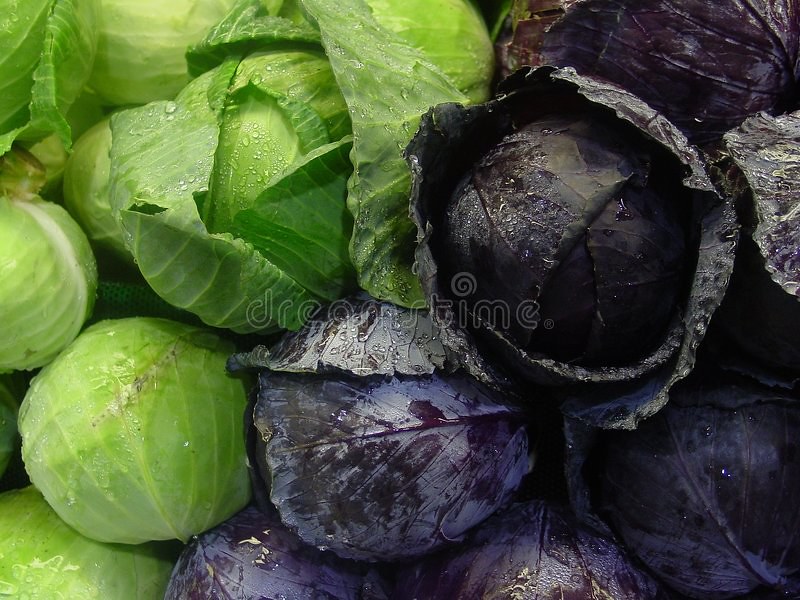A vivid, close-up colour photograph captures an artful arrangement of fresh cabbages in a landscape orientation. The image features two types of cabbages—green on the left and shades of purple, almost black, on the right—forming a visually striking collage. The green cabbages cascade diagonally from the lower left-hand corner up towards the center, creating a lush, leafy foundation. In contrast, the right side is dominated by tightly wound, spherical purple cabbages, with some leaves partially open, adding textural variety. Droplets of what could be rainwater or humidity glisten on a few leaves, enhancing the freshness of the scene. Superimposed faintly in the center of the photograph is the text "dreams time" in a delicate white lowercase font, with a whimsical swirl dotting the 'i'—lending a dreamlike quality to the meticulously stacked display, reminiscent of a market's produce section.